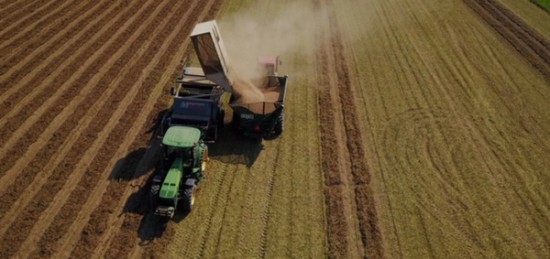The photograph is a detailed aerial view of a farming field showcasing two tractors engaged in an agricultural operation. The prominent tractor, colored green and identified as possibly a John Deere, is positioned just to the left of the image’s center, facing downward with its hood towards the bottom of the frame. Attached to its back, it pulls a machine fitted with a hydraulic lift, which is actively tilting a box to pour grain. The grain cascades into a large receiving basket on the front of a second tractor situated to the right. Plumes of smoke or dust rise as the grain is deposited. The field itself shows clear signs of recent activity: the left side displays neatly tilled soil while the right side still retains green vegetation, untouched by the agricultural process currently underway. The tractors move in parallel rows, with the right tractor slightly trailing to efficiently collect the harvested grain.